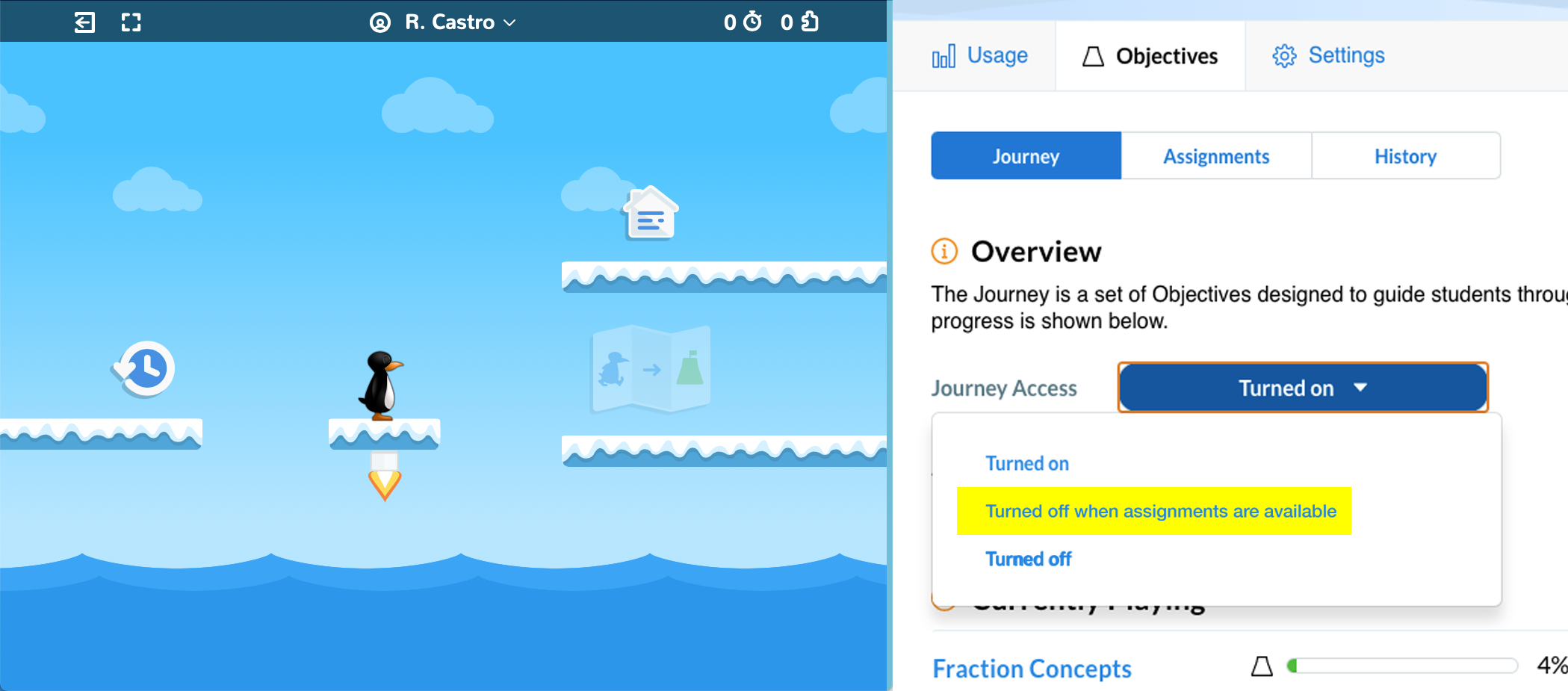The image consists of two desktop windows displayed side-by-side.

**Left Window:** 
- **Header Features:** There's a menu bar at the top featuring an exit button, a zoom-in option, and a user profile labeled "r.castro" with a drop-down menu. Additionally, it shows icons indicating "0," a timer, another "0," and a puzzle piece.
- **Game Interface:** The scene resembles a game set within a blue ocean backdrop, under a sky adorned with clouds. The aesthetics are cartoon-like. The scene features several platforms, four in total, with blue coloring and white ice caps.
  - **Game Elements:**
    - A clock above one of the platforms counts down time.
    - A cartoon penguin stands on a small platform, indicated by an orange downward-pointing triangle beneath it.
    - To the right of this platform is a larger platform with an illustration of the penguin running towards a distant green mountain.
    - At the highest platform, there’s an image of a house.

**Right Window:** 
- **Preferences Screen:** This window seems to be part of a preferences or settings menu.
  - **Categories and Icons:** It lists various sections such as "Usage" (marked by a bar graph), "Objectives" (depicted by a bell icon), and "Settings" (denoted by a cogwheel).
  - **Highlighted Sections:** The "Journey" section is highlighted with a blue square and white text, while "Assignments" and "History" are indicated with white squares and blue text.
  - **Information Icon:** An orange information icon appears with the label "Overview" beside it.
  - **Details:** The description mentions, “The journey is a set of objectives designed to guide students through progress, as shown below, journey access.”
  - **Toggle Button:** There is a toggle switch highlighted in red, currently set to "Turned On," with options for "Turned Off when assignments are available" (highlighted in yellow) and a simple "Turned Off" option.
  - **Progress Information:** Below these settings, a section labeled "Fraction Concepts" shows that progress is only at 4%, indicating the educational nature of the software.
  - **Blocked Content:** A pop-up message partially blocks the content below, which appears to include the text "currently playing."

This setup suggests an educational edutainment software designed to engage students in learning activities, combining game-like elements with progress tracking and educational objectives.